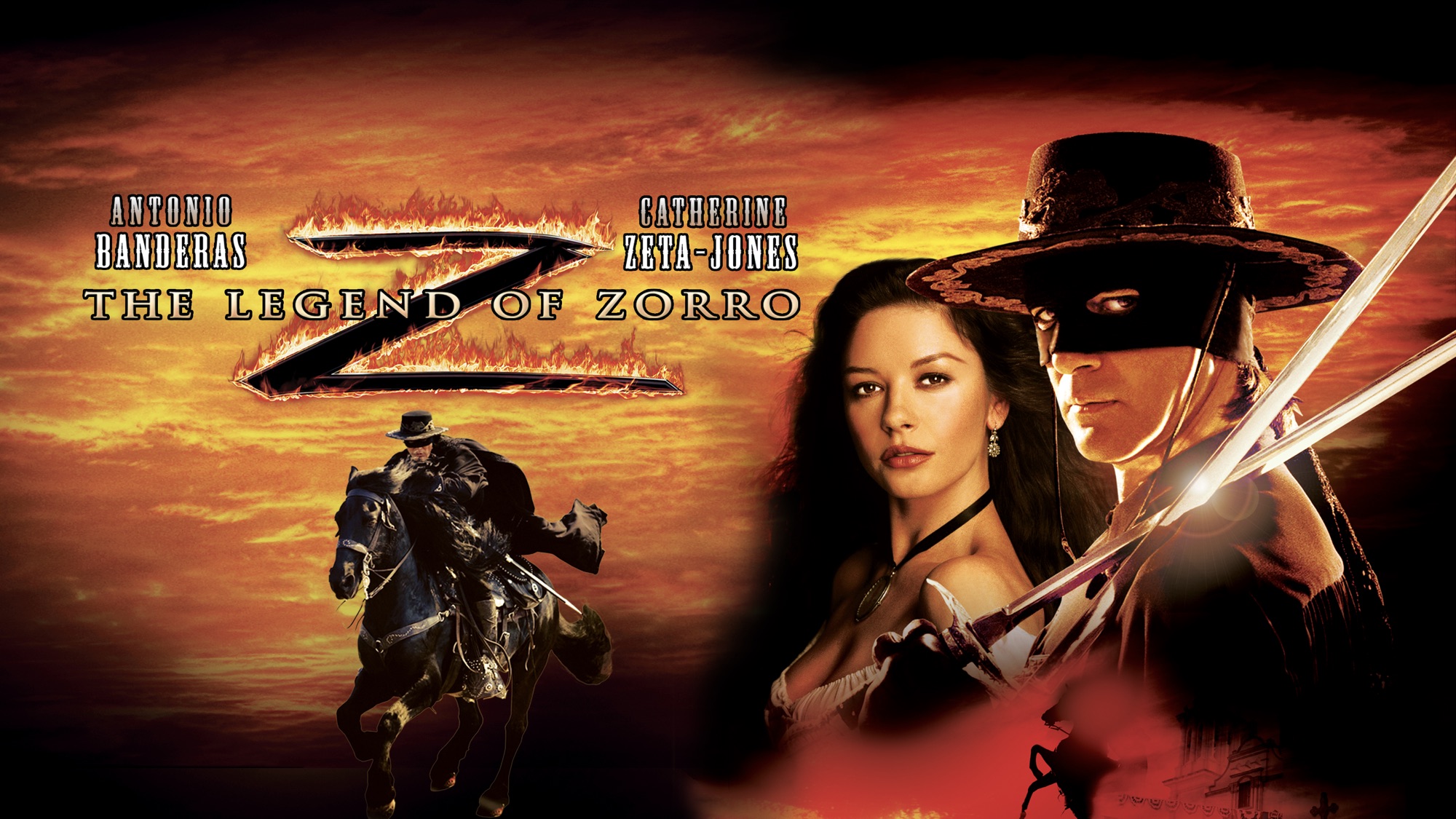This vibrant and fiery promotional image for "The Legend of Zorro" showcases a dynamic scene drenched in shades of orange and golden yellow, reminiscent of fire. Dominating the scene on the left side, we see the title "The Legend of Zorro" emblazoned with a striking, flaming letter Z in the background. Below the title, Antonio Banderas, in character as Zorro, is depicted in his signature black attire, complete with a black cape, wide-brimmed hat, and a black mask, as he rides a galloping white horse. 

On the right side of the image, there's a dramatic close-up of Antonio Banderas and Catherine Zeta-Jones. Zorro, still clad in black and wearing his distinctive eye mask, stands with a sword resting casually over his left shoulder, his intense gaze fixed on the viewer. Beside him, Catherine Zeta-Jones, with her lush, long dark hair cascading below her chest, and dressed in a low-cut outfit adorned with earrings and a black necklace, also directs a charming yet fierce look towards the camera. Their swords are crossed in a poised stance, symbolizing their strong and determined characters. The actors' names, "Antonio Banderas" and "Catherine Zeta-Jones," hover prominently above them, accented by the fiery Z of Zorro, capturing the essence of adventure and romance that defines the movie.